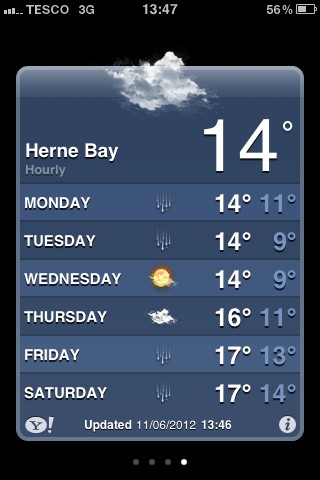This is a detailed smartphone screenshot displaying a weather summary. The top section of the screen features a black background transitioning to light gray. In the top-left corner, the signal strength indicator reads "Tesco" and "3G." The center showcases the time, "13:47", while the top-right corner displays the battery level at 56%.

Below this, a predominantly blue and dark blue portrait-style rectangle presents the weather details. At the top of this rectangle, a dark and gray cloud icon signifies the current weather condition. Directly beneath, it indicates the location, "Hearn Bay", with "Hourly" noted underneath. A large white numeral displays the temperature as 14°C.

The forecast for the next six days follows, each day on its individual color-bar. The bars alternate between lighter blue and darker blue backgrounds. The days of the week are written in white, capitalized text:
- Monday: Light blue bar with a rain symbol. High 14°C - Low 11°C.
- Tuesday: Dark blue bar with a rain symbol. High 14°C - Low 9°C.
- Wednesday: Light blue bar with a partly sunny symbol. High 14°C - Low 9°C.
- Thursday: Dark blue bar with a cloud symbol. High 16°C - Low 11°C.
- Friday: Light blue bar with a rain symbol. High 17°C - Low 13°C.
- Saturday: Dark blue bar with a rain symbol. High 17°C - Low 14°C.

The bottom-left corner of the weather block features the Yahoo logo, a circle with a "Y!" inside it. "Updated 11/06/2012 at 13:46" is noted in the center. The bottom-right corner contains an info icon, a circle with an "i."

Lastly, at the bottom of the screen, four dots are displayed, indicating multiple screens available within the app. The one white dot suggests this is the current visible screen, while the other three are gray.